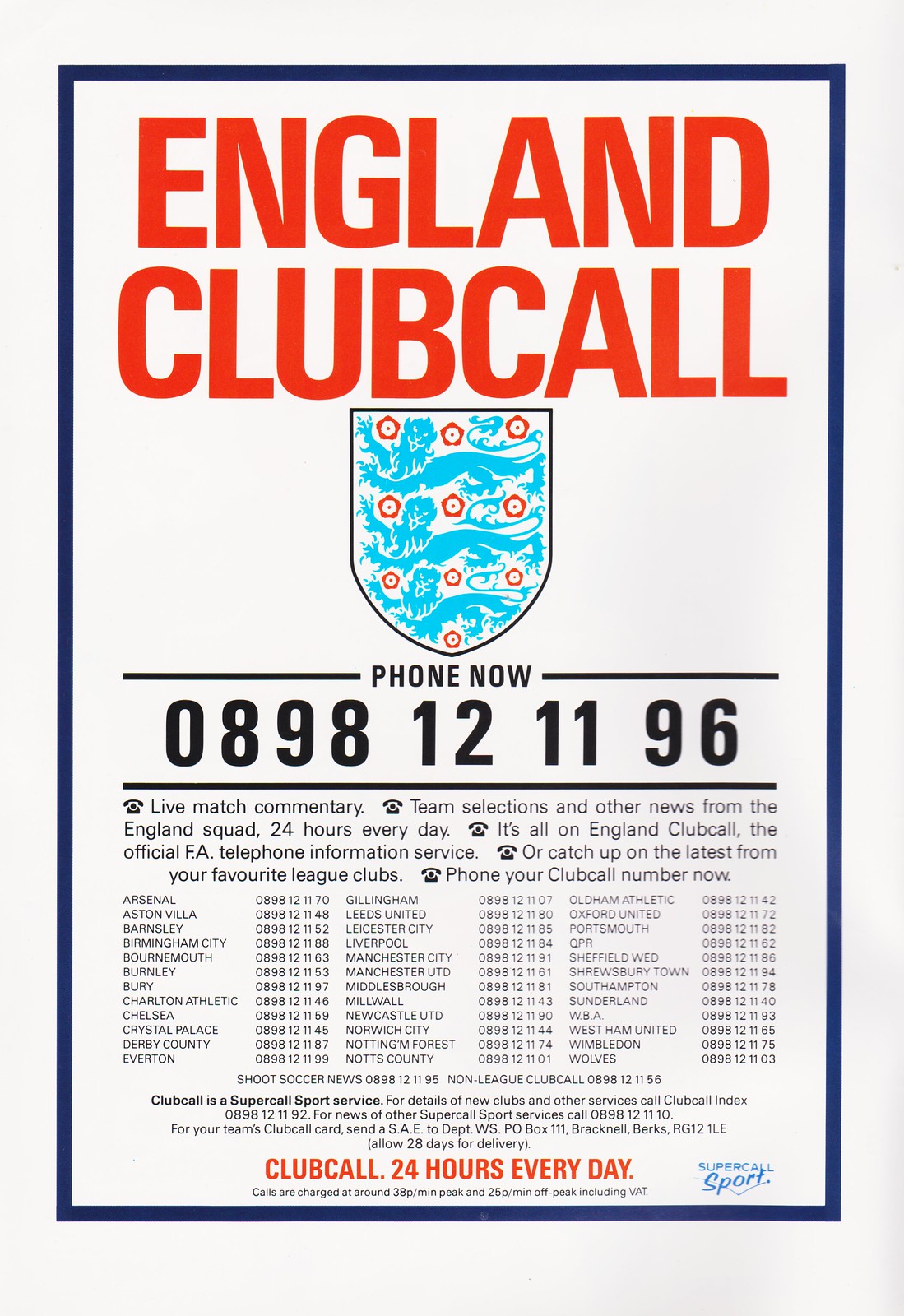The image depicts a detailed poster advertising England Club Call, an official FA telephone information service providing live match commentary, team selections, and other news from the England squad and various league clubs 24 hours a day. The poster features a thin navy blue rectangular border surrounding it, with bold red text at the top announcing "England Club Call." Beneath this heading, a shield logo containing an image of a blue dragon and red flowers is prominently displayed. Directly below the shield, the text "Phone now: 0898 121 196" is written in bold black font, inviting viewers to call for the latest updates.

The poster further elaborates on the offerings of England Club Call, stating: "Live match commentary, team selections, and other news from the England squad, 24 hours every day. It's all on England Club Call, the official FA telephone information service. Or catch up on the latest from your favorite league clubs. Phone your club call number now." Below this, a comprehensive list of football clubs and their respective contact numbers follows, including:

- Arsenal 0898121170
- Aston Villa 0898121148
- Barnsley 0898121152
- Birmingham City 0898121888
- Bournemouth 089812163
- Burnley 08981253
- Bury 08981297
- Charlton 08981246
- Chelsea 08981259
- Crystal Palace 08981245
- Derby County 08981287
- Everton 08981299
- Gillingham 08981207
- Leeds United 08981280
- Leicester City 08981285
- Liverpool 08981284
- Manchester City 08981291
- Manchester United 08981261
- Middlesbrough 08981281
- Millwall 08981243
- Newcastle United 08981290
- Norwich City 08981244
- Nottingham Forest 08981274
- North Country 08981201
- Oldham Athletic 08981242
- Oxford United 08981272
- Portsmouth 08981282
- QPR 08981262
- Sheffield Wednesday 08981286
- Shrewsbury Town 08981294
- Southampton 08981278
- Sunderland 08981240
- WBA 08981293
- West Ham United 08981265
- Wimbledon 08981275
- Wales 08981203

Other services mentioned include Shoot Soccer News and Non-League Club Call, with contact numbers 0898121195 and 0898121156 respectively. Additional information on super-call sports services and details for obtaining a club call card via mail are provided, including charges of 38 pence per minute at peak and 25 pence per minute off-peak. The poster concludes with the tagline "Club Call 24 hours every day," and features the Super Call Sport logo at the bottom right corner.